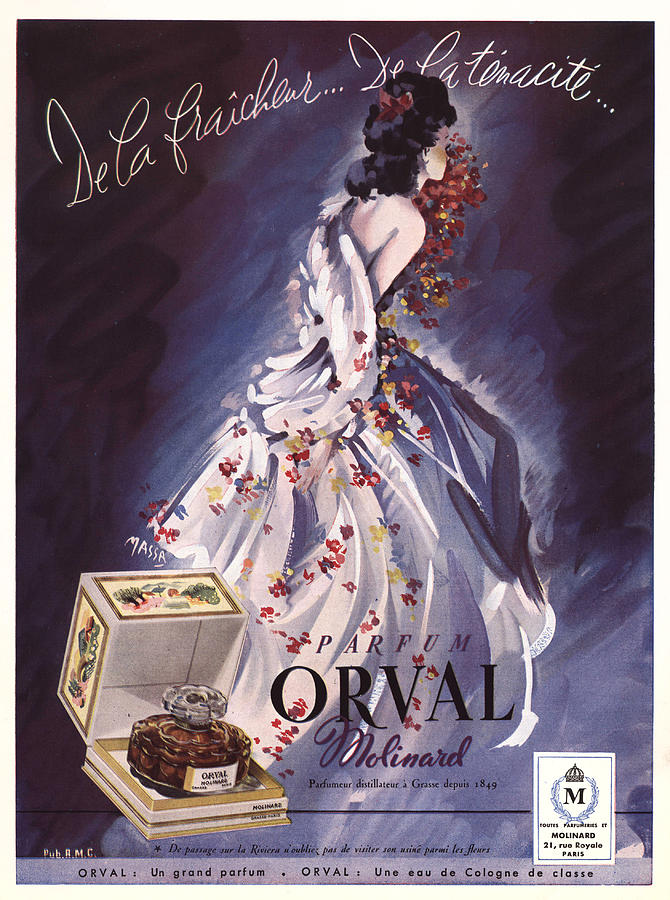This vintage French perfume advertisement, likely from the 19th century, features a detailed illustration with a captivating aesthetic. At the top of the ad, cursive script arcs to present the names "De La Fresiere, De La Tenisipe." Central to the image is an elegant woman with an intricate, black updo adorned with a small red butterfly-like ribbon. She wears a luxurious white swan-like shawl over a stunning white ball gown, exuding an ethereal charm. Her face is turned slightly, revealing only the tip of her ear and one eye, while her one bare shoulder peeks out beneath the shawl. 

The background of the image transitions from a rich, dark purple to a lighter purple and blue gradient, finally highlighting the figure with a soft white glow. Surrounding the woman is a cascade of flower petals, beginning near her face and loosely trailing across her dress. Prominently displayed near the bottom of the ad is a beautifully decorated box containing the Orval Malenard perfume glass bottle, with the perfume name "Parfum Orval Malenard" inscribed nearby. Additional text at the bottom reads "Parfumer Distillateur à Grasse Depuis 1849," emphasizing the fragrance's heritage. The composition is accented by the Malenard logo situated in the lower right corner, completing the sophisticated and visually engaging advertisement.